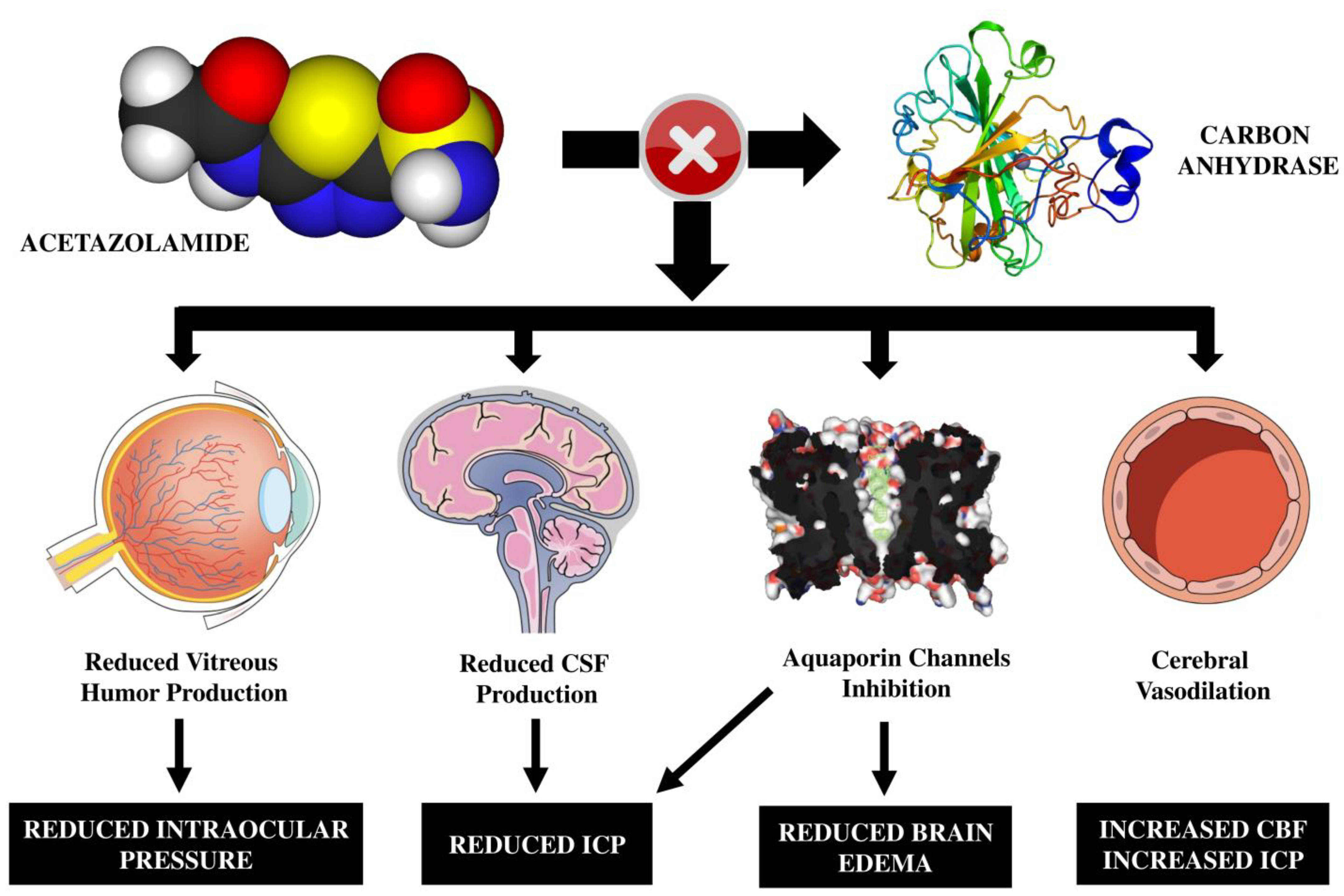The image is a detailed science diagram divided into two levels, both filled with descriptive text and illustrations. Black arrow marks guide the progression through the diagram. In the center, a red circle encloses a prominent X mark. 

To the top left, there is a molecular cluster labeled acetazolamide, depicted with yellow, blue, red, and white spherical structures. On the right side, there is a coiled structure named carbon anhydrase, featuring green, blue, red, and yellow elements.

The central layer of the image includes several key biological processes represented by various illustrations. Firstly, an eyeball is labeled "reduced vitreous humor production, reduced intraocular pressure." Next, the brain is shown with the text "reduced CSF production, reduced ICP" beside it. Adjacent to the brain, there is a depiction of aquaporin channel inhibition or reduced brain edema, illustrated with brownish, green, and pink shapes. To the far right, cerebral vasodilation is symbolized by a pink circle and is annotated with "increased CBF and increased ICP."

This infographic effectively conveys complex relationships between different body parts and chemical interactions.